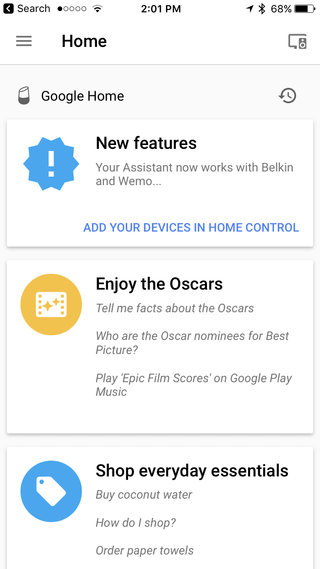A detailed screenshot from a smartphone displays various components of a home automation assistant interface. 

At the very top, the status bar indicates the current time, 2:01 PM, along with the battery level at 68%, and the word "Search" on the left. Directly below, a navigation bar shows "Home."

The main section features a grey background with three white rectangular boxes. The first box, highlighted with a blue exclamation mark on its left, announces "New Features" and informs the user that their assistant now integrates with Belkin and Wemo. Below this, in bold blue capital letters, it prompts the user to "ADD YOUR DEVICES AND HOME CONTROL."

The second box features an orange circle with a white design, conveying entertainment options related to the Oscars. It includes prompts such as "Enjoy the Oscars," "Tell me facts about the Oscars," "Who are the Oscar nominees for Best Picture," and "Play epic film scores on Google Play Music."

The third box is distinguished by a blue circle bearing a white price tag icon. This section focuses on shopping for everyday necessities, containing commands like "Shop everyday essentials," "Buy coconut water," "How do I shop," and "Order paper towels."